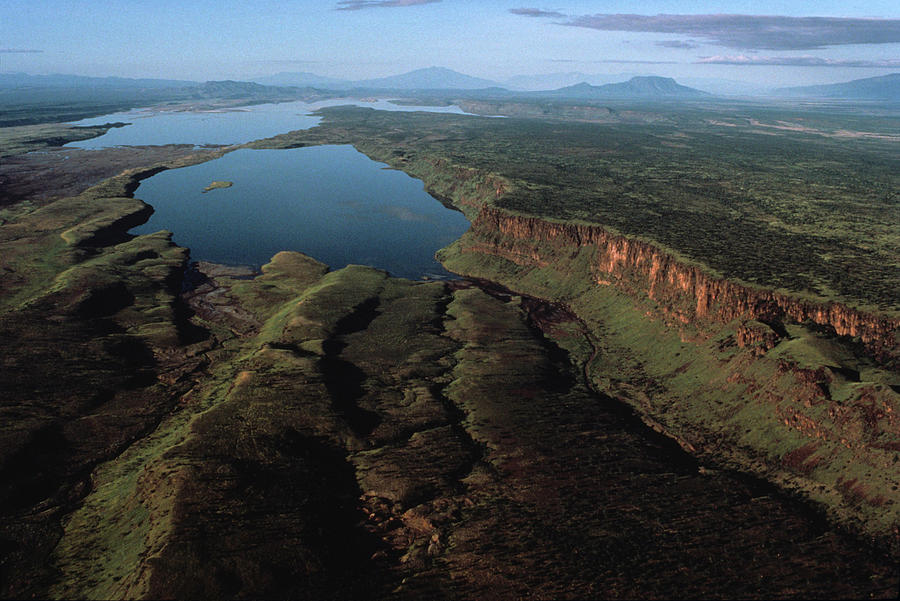This is an expansive aerial photograph capturing the wild, untamed beauty of a vast, fjord-like landscape. Central to the scene are two large, deep blue lakes of varying shapes that reflect the sky above, giving them a serene appearance. These lakes are seamlessly interconnected, nestled within craggy, green terrain dotted with patches of brown dirt and reddish, clay-colored rocks. The rugged terrain is richly covered in moss and other greenery, showcasing the untouched nature of this picturesque landscape. 

The midground features rocky formations, some steep cliffs with striking red clay, especially noticeable on the right-hand side, which give way to further greenery at their peaks. As the terrain stretches towards the horizon, the scene is enveloped by a chain of towering mountains partially veiled in fog and adorned by scattered clouds. The sky is a brilliant blue, punctuated by wisps of gray and white clouds, contributing to the majestic and seemingly endless view. The photograph emphasizes the natural grandeur and solitude of the location, entirely devoid of human presence, highlighting the pristine, raw beauty of this remote wilderness.